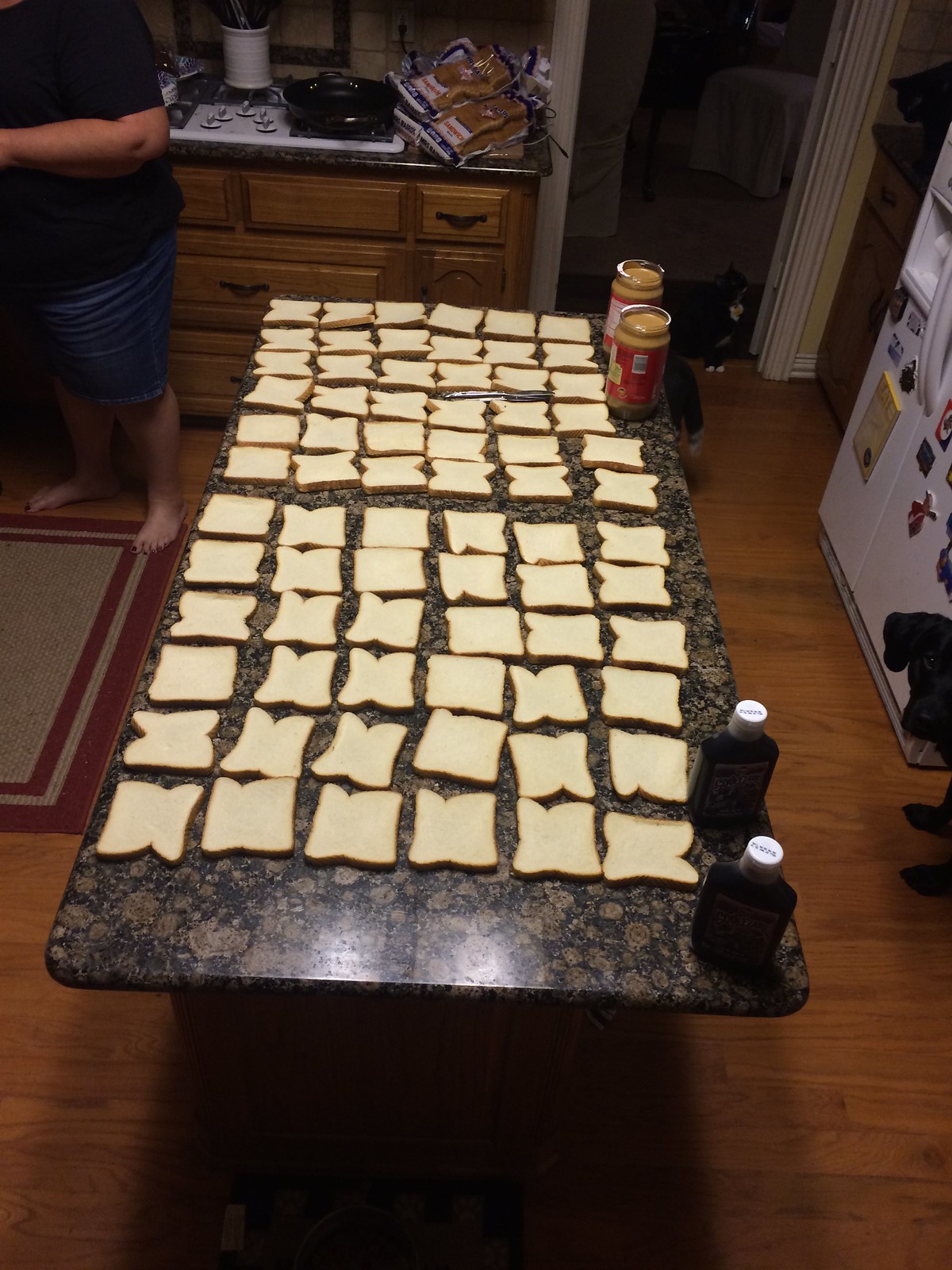The image is a color photograph taken from above, showcasing a granite kitchen island meticulously prepared for making sandwiches. Laid out on the island are 72 slices of white bread, arranged neatly in a grid of 12 rows and 6 columns. Behind the bread, there are two large jars of peanut butter with red labels, and on the right side of the island, two large squeeze bottles of grape jelly are visible. The preparations suggest an endeavor to make peanut butter and jelly sandwiches, possibly for a picnic or a charitable cause such as feeding the homeless.

In the foreground, a part of the kitchen floor is visible, which is made of either laminate or hardwood. The right side of the photo features a black dog with just its ear, nose, and front paws in view. Also partially visible is the lower part of a white refrigerator adorned with magnets. In the upper right corner, a narrow doorway can be seen, with a black and white cat sitting in it. The background includes lower kitchen cabinetry and more countertop space cluttered with various items. 

A person, possibly a woman, is partially cropped out of the photo. They are wearing a dark shirt, jean shorts, and are barefoot, standing on a tan kitchen rug with red-striped borders. The overall scene captures a moment of careful preparation and organization for a generous endeavor in a well-used kitchen.